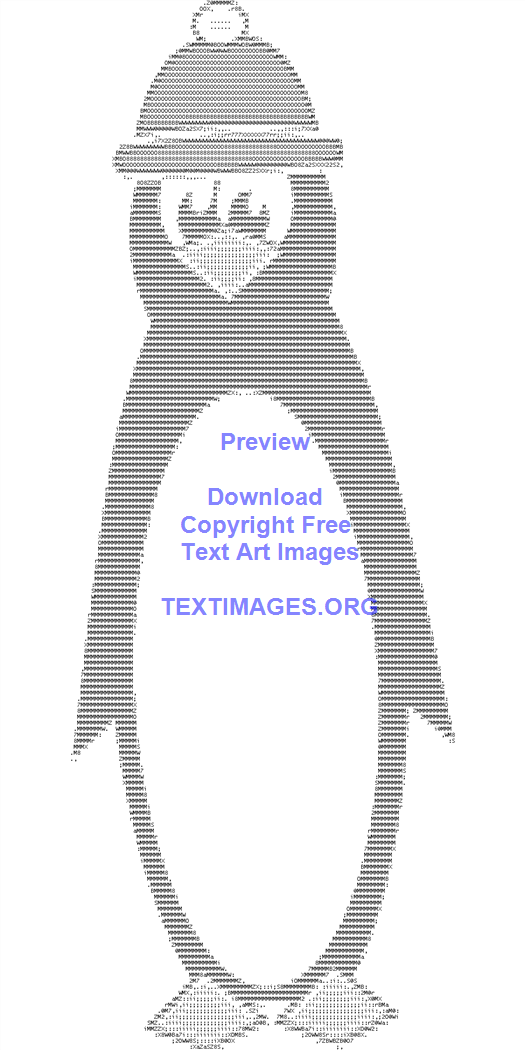This detailed ASCII art illustration features a tall, skinny cartoon penguin meticulously crafted from typed characters. The penguin's body, including the white oval belly, is formed by carefully arranging letters and characters, with the negative space contributing to its clean outline. The penguin sports a toboggan-style beanie, complete with a rolled-up brim and a white pom-pom on top, adding a whimsical touch. Its large googly eyes and small triangular beak give it an engaging expression as it looks directly at the viewer. The artwork is accompanied by a blue watermark in the center that reads, "Preview. Download copyright-free text art images at textimages.org."